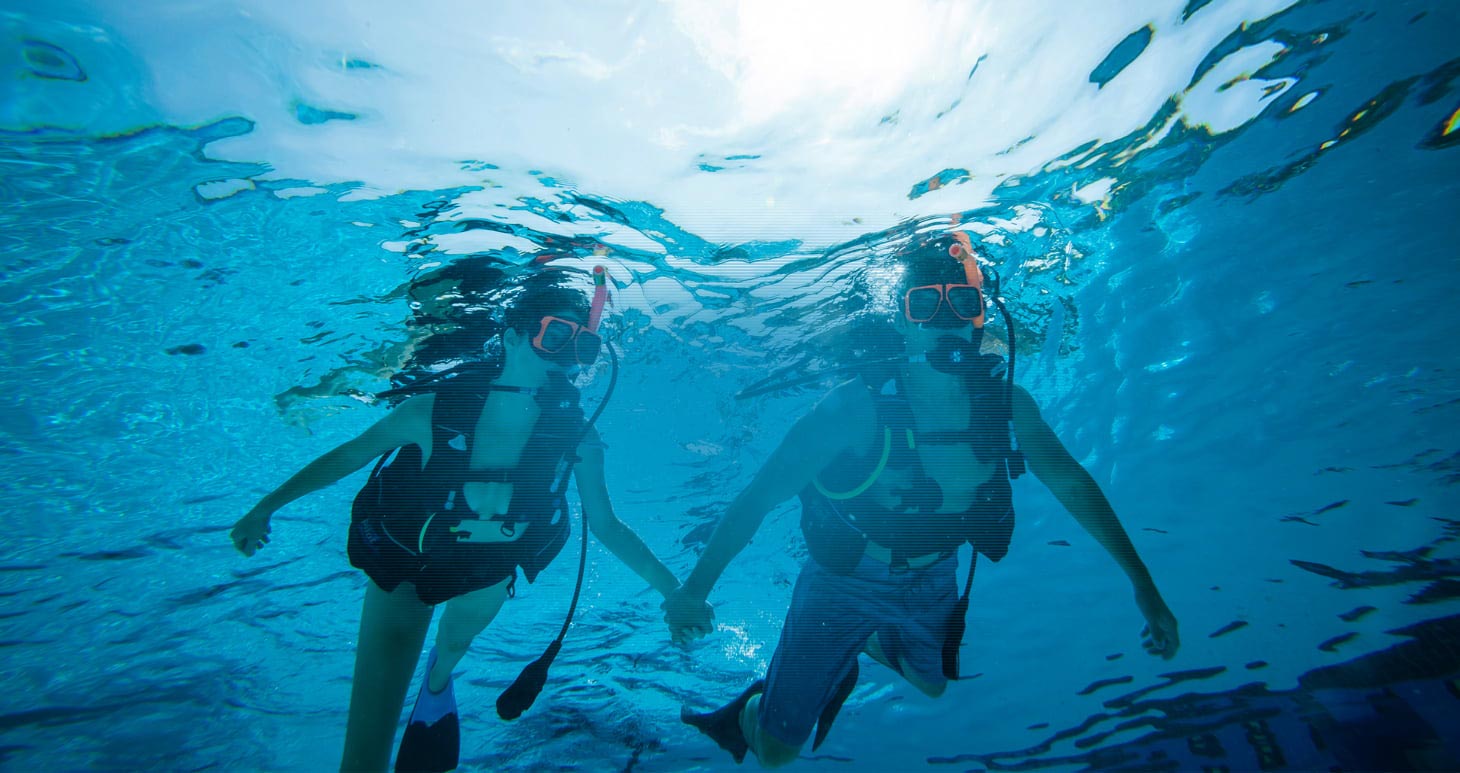In this captivating underwater photograph, we see a couple snorkeling in crystal blue waters. The image captures the man and woman from below as they float near the surface, their bodies fully visible. Both are wearing snorkeling gear, including large goggles and orange snorkel tubes that extend above the water. They are holding hands, and their swim attire includes black vests supporting their tanks, long swim pants, and black swim fins. The woman, on the left, has her right leg bent at the knee, while the man, on the right, mirrors this pose. Above them, sunlight filters through the water, creating a bright white circle in the top center and illuminating the scene with varying shades of blue and white, indicative of water movement. The sandy ocean floor with scattered dark particles is faintly visible below. There are no fish in the visible area of the shot, ensuring that the focus remains on the couple's intimate snorkeling experience.